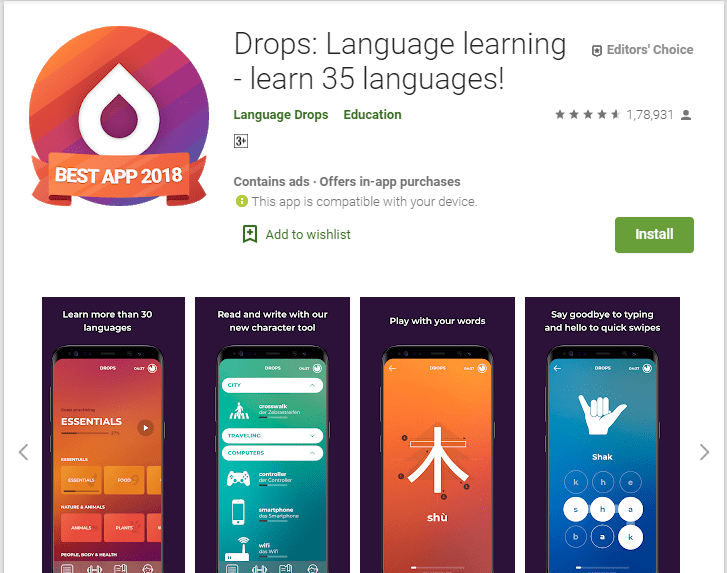Image Description:

The image has a predominantly white background. In the upper left-hand corner, there's a circular gradient ranging from very light orange at the outer rim to a darker orange, red, purple, dark blue, and gradually transitioning into lighter shades of blue toward the center. Inside this circle, there's a white teardrop or raindrop shape.

Beneath the circle is an orange and white banner reading "Best App 2018."

On the right-hand side, the text "Drops Language Learning" is displayed prominently, followed by "Learn 35 languages" written in green. Below this, additional information reads "Language Drops Education," "3+," "Contains ads," "Offers in-app purchases," and "This app is compatible with your device." In green text, there is an "Add to Wish List" option.

On the upper right side, there is an "Editor's Choice" badge, followed by four and a half gray stars and the number "1,873,391," indicating the number of reviews.

At the bottom right, there's a green "Install" button with white text.

Below this button, there are four screenshots from the app, each featuring white text at the top. The first screenshot says "Learn more than 30 languages with our new character tool." The second and third screenshots are not described. The fourth screenshot says "Say goodbye to typing and hello to quick swipes." The screenshots have varied background colors: yellow, blue, yellow, and blue, respectively.

That's all!